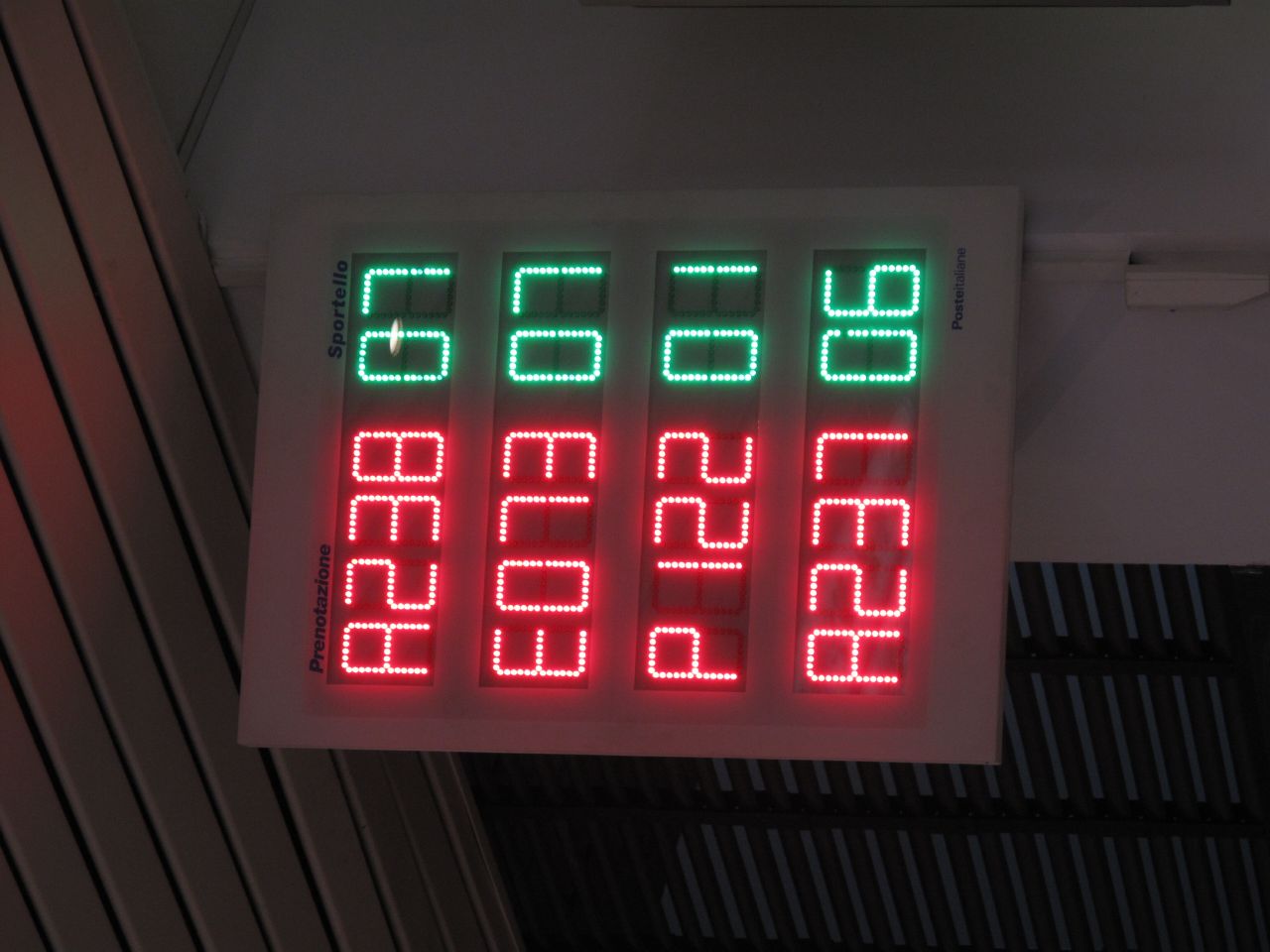The photograph captures a rectangular, vertically oriented LED sign mounted on a white building, with a black gate to the left. The sign is illuminated amidst a dim, possibly nighttime setting. The top of the sign is marked by two headings: "Prenotaziano" on the left in black text and "Sportello" on the right, also in black. Below these headings, the sign features four rows of LED lights displaying a combination of letters and numbers. Each row consists of red alphanumeric characters on the left and green numbers on the right. 

The first row reads "A238" in red with "07" in green;
The second row displays "E073" in red next to "07" in green;
The third row shows "P122" in red alongside "01" in green;
The fourth and final row lists "A237" in red with "06" in green.

Each character is formed by small light circles, contributing to the glowing appearance of the sign amidst the dark surroundings.